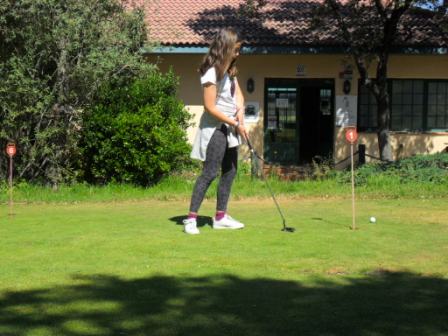The photograph, slightly out of focus likely due to a low-quality camera, captures an outdoor scene bathed in warm, bright sunlight. Central to the image is a young girl practicing mini-golf on a grassy yard. She has shoulder-length brunette hair and is dressed in a white t-shirt, black leggings, and white tennis shoes. The girl's putter is poised over a golf ball that has rolled just past a hole marked by a short pole with an orange disc bearing the number one. Nearby, another similar hole with an orange disc is visible.

In the background stands a yellow building with dark windows and a terracotta roof partially shadowed by a tree to the right. Additional greenery, including some shrubbery on the left and lush, green grass underfoot, enhances the summery outdoor ambiance. The sun casts defined shadows on the ground, suggesting that the scene is shaded by a tree above or near the photographer.